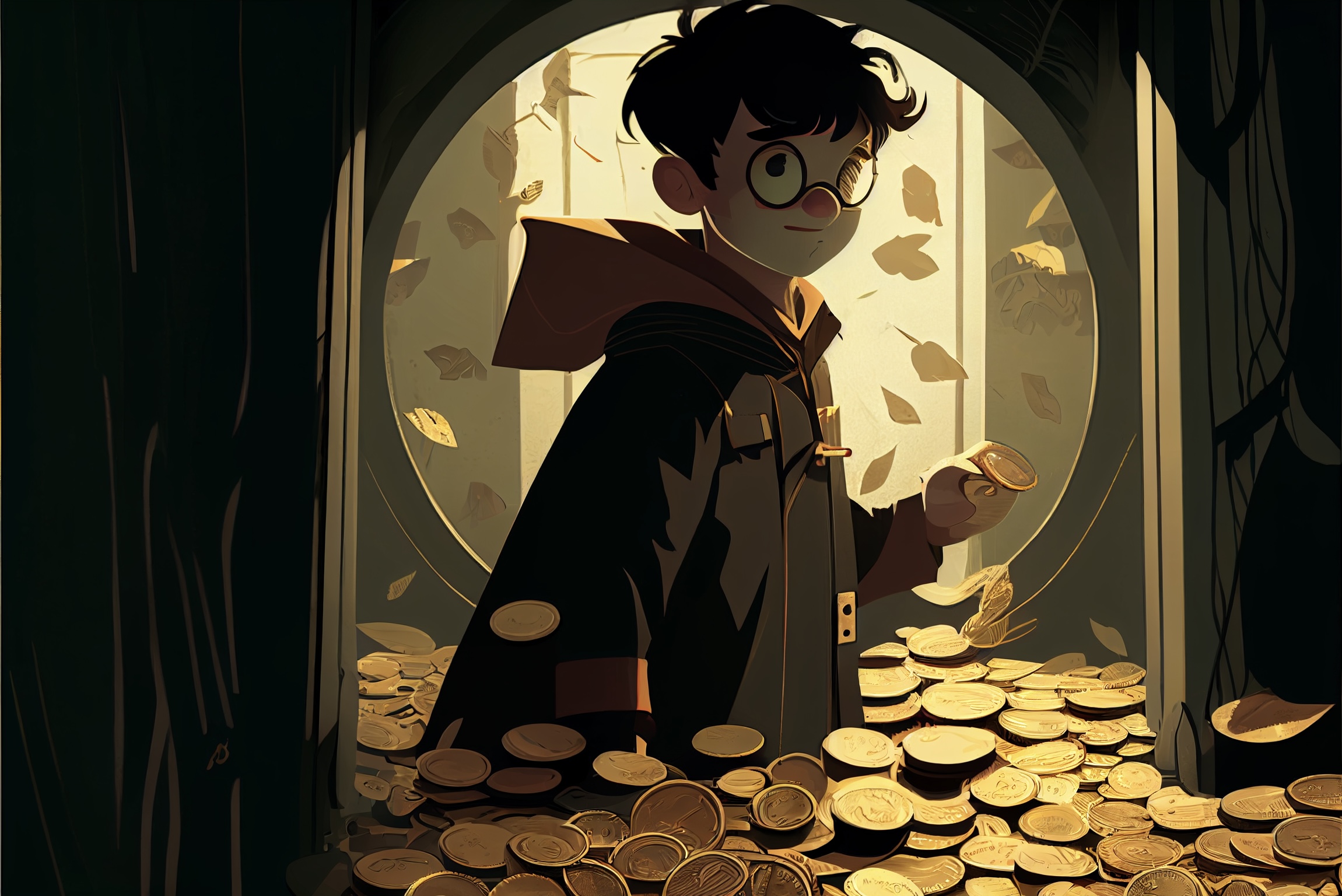The image is an animated drawing featuring a boy who resembles Harry Potter. He stands waist-deep in a large pile of gold coins, with an expression that includes a smirk. The boy, who has disheveled black to brown hair and big ears, is wearing round glasses which accentuate his striking red nose. He is dressed in a dark parka-like jacket with a hood that is down at the back. The jacket is primarily black with red trim details at the cuffs and hood, and it appears to be zipped up. The background shows a somber, dusk-like setting with dark blacks, browns, golds, and reds dominating the color palette. There is a circular window behind him through which leaves are falling. Additionally, there are wood panels framing the scene to the left and right, lending a rustic feel to the environment. The boy holds a coin in one hand, emphasizing the wealth surrounding him, while the overall atmosphere is muted and mysterious.